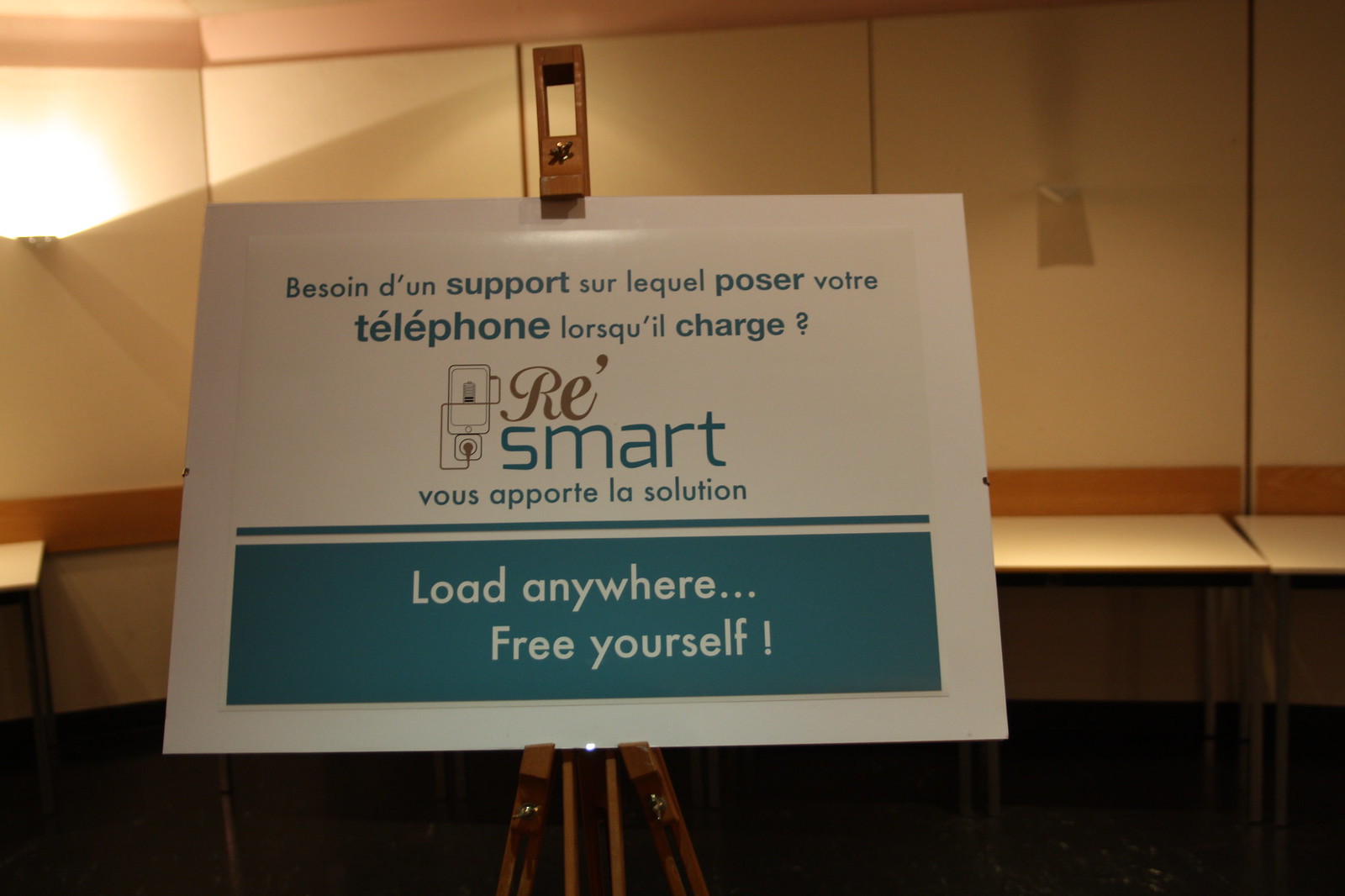The photograph captures a sign on a wooden easel inside what appears to be a presentation or conference room. The sign itself is predominantly white with a blue line at the bottom and contains text in a language that resembles French, along with some English words. The primary text reads "Besoen d'un support sur l'equel poser votre téléphone lorsqu'il charge," followed by "reSmart vous apportez la solution." Prominently in the center of the sign is an image of a phone being plugged into the wall, and next to it, the word "SMART" is visible. At the bottom of the sign, in white letters against a blue background, the phrase "LOAD ANYWHERE FREE YOURSELF!" stands out. 

The background reveals beige walls with a wooden rail and several white tables lined up against the wall. Warm lighting fixtures are affixed to the wall, contributing to a cozy ambiance. The room seems well-arranged, likely intended for a formal gathering or presentation.